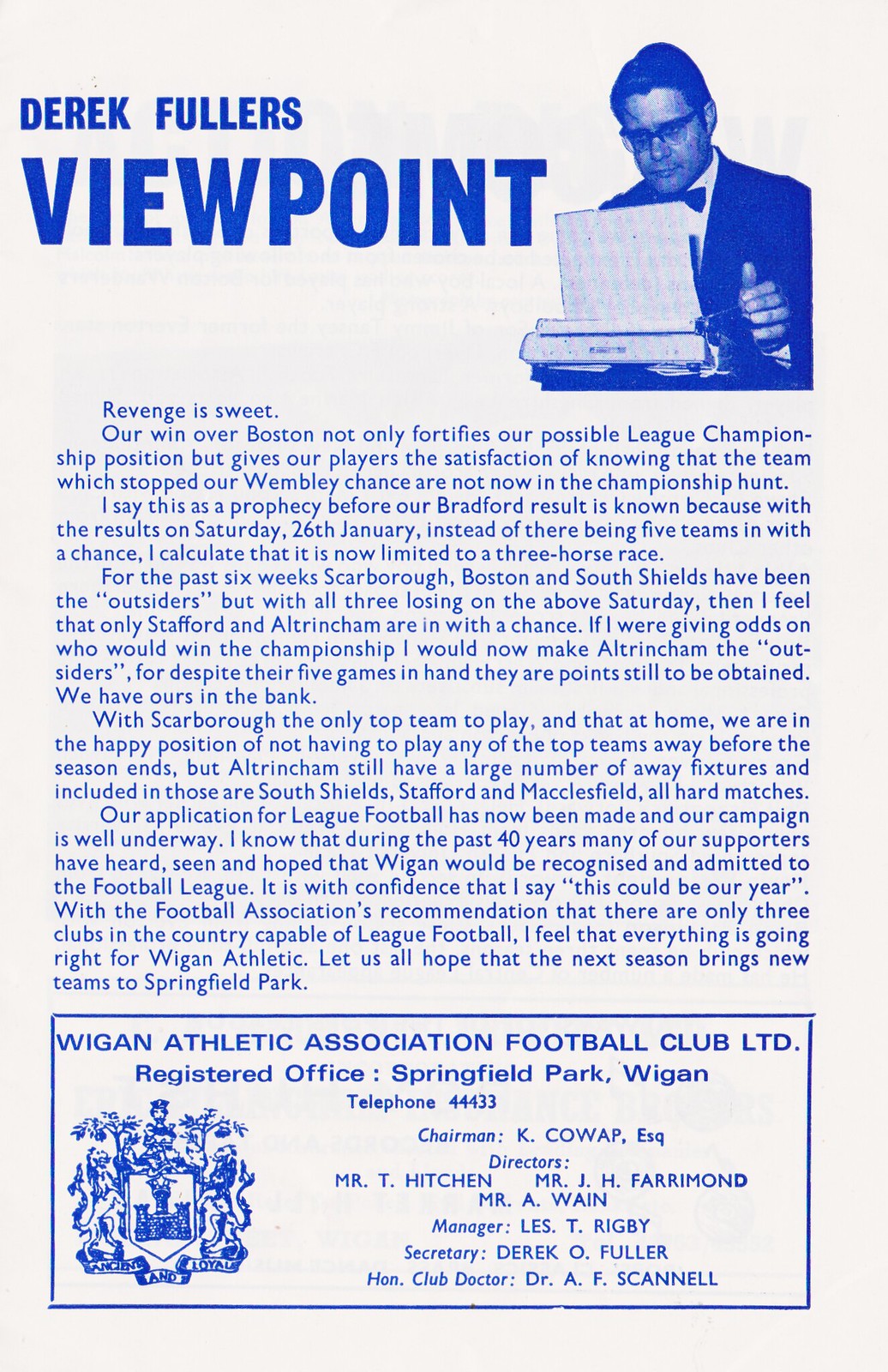The flyer titled "Derek Fuller's Viewpoint" is presented on an ivory-colored paper with all text in a royal blue font. The title "Derek Fuller's Viewpoint" is left-aligned, accompanied by a photograph of a bespectacled man working at a typewriter on the right. The article opens with the header "Revenge is Sweet" and goes on to recount a satisfying victory over Boston, stressing its importance for the league championship race. The text details Derek Fuller's prediction of the championship competitors, mentioning teams such as Scarborough, Boston, and South Shields, and focusing on the potential contenders Stamford and Altrincham. At the bottom third of the flyer, a boxed section contains information about the Wigan Athletic Association Football Club, Ltd, including the registered office at Springfield Park, Wigan, telephone number 44433, and names of the chairman, directors, manager, secretary, and the honorable club director. A logo representing the football club is positioned on the bottom left of the flyer.